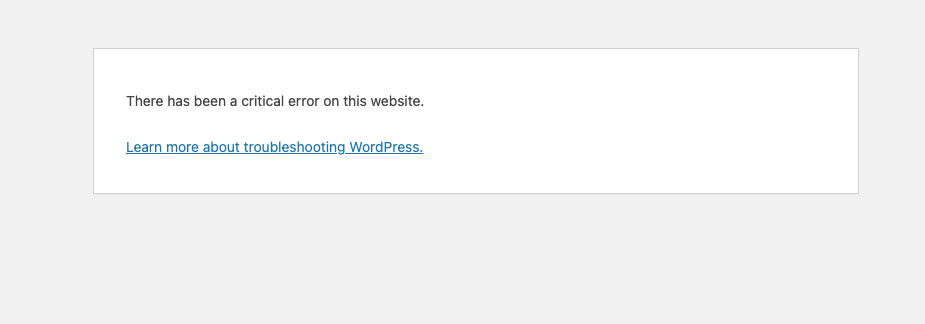This image shows a simplistic landing page, suggesting a malfunction on the website. Captured from a laptop, desktop, smartphone, or tablet, the background is a dark gray. Towards the left side, centrally positioned, there is a light gray rectangle. Inside this rectangle, in black text, the message reads, "There has been a critical error on this website." A period follows this sentence. Below it, in new, hyperlinked blue text, the message "Learn more about troubleshooting WordPress" appears, underlined. The light gray rectangle has a border on all sides. The image appears to be cut off, so there are no additional details visible.